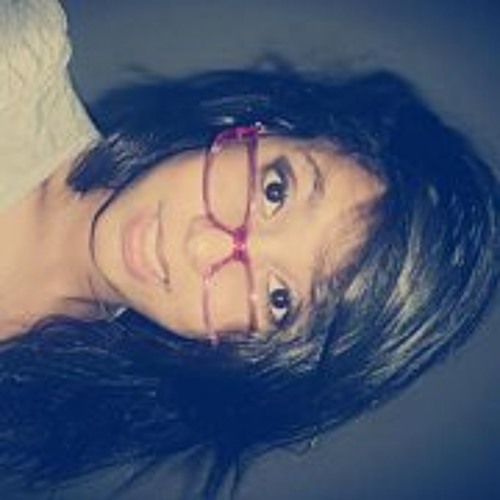This is a detailed headshot of a young woman with shiny, shoulder-length black hair against a dark gray background. The woman's head is turned sideways, so her face appears horizontally across the image with the top of her head on the right and her neck on the left. She’s wearing a pair of pink or purple reading glasses (stated as red in one description), complementing her brown eyebrows and eyes (described as either brown or black). She is smiling gently, revealing a blurred glimpse of her teeth. The attire she's wearing is a white top, possibly a blouse or a sweater, with a V-neck or U-neck style. The overall expression exudes a warm and friendly demeanor. Based on the features described, she could be either Hispanic or Asian.